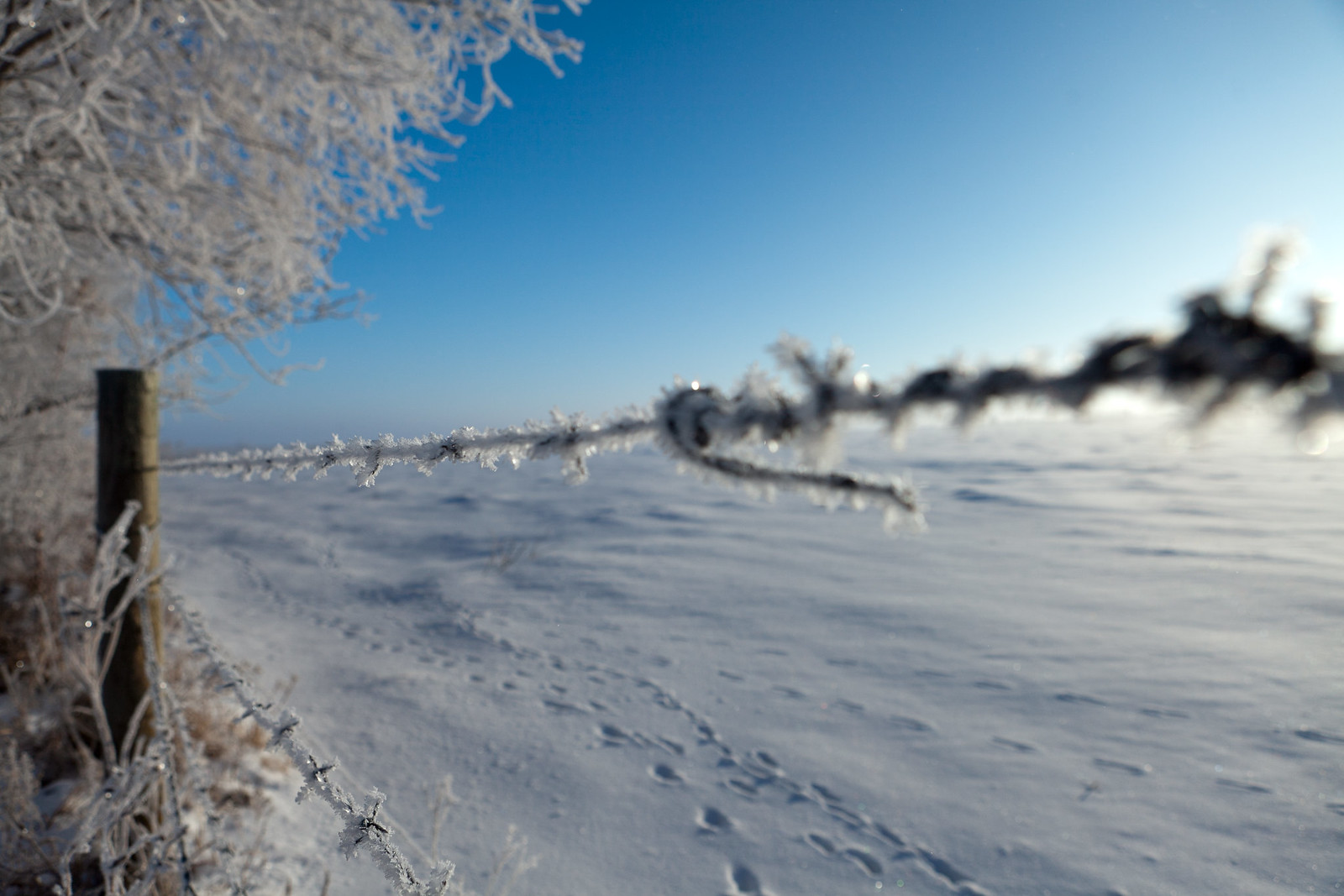This detailed image is a color photograph capturing a stark and serene winter scene. The foreground features a wooden fence post to the left, adorned with a barbed wire fence that's heavily frosted and encrusted with ice. The ice-covered wire stretches horizontally across the frame, leading the eyes toward the snowy expanse beyond. The ground is blanketed in pristine, untouched snow, except for a few deer and human footprints that meander through the open field, adding a touch of life to the still landscape.

To the left side of the image, there's a mix of shrubs and a large tree. The tree's limbs are heavy with snow and ice, each branch outlined sharply against the bright blue sky. In the background, the snowy terrain extends all the way to the horizon, which bisects the photograph horizontally, accentuating the vastness of the scene. The sky above is a radiant, clear blue, fading to almost white on the right side of the picture, suggesting the sun's presence and adding a subtle gradient to the sky's color.

Overall, the scene depicts a crisp, cold winter day in an open, snowy field watched over by frozen trees and a silent fence, all bathed in the clarity of daylight. The image has a unique and tranquil beauty, juxtaposing the cold harshness of winter with the serene calm of the natural landscape.